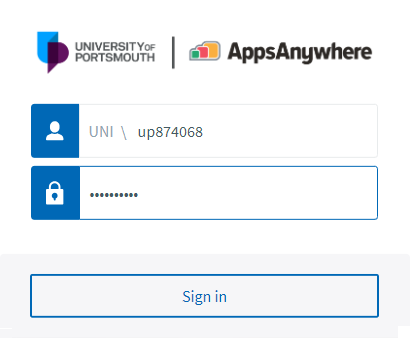This image features a clean, white background and presents a screen page with detailed elements. At the top left corner, there is a logo that includes a unique blue object resembling a U-shaped shield. To its right is a dark purple element that bears resemblance to the letter P. Adjacent to these elements, the text reads "University of Portsmouth." 

Below this, a thin vertical black line separates three small squares, colored green, red, and orange respectively. This section is labeled "Apps Anywhere."

Further down, there is a box displaying a blue square on the left side with a generic profile picture. Next to this image, text reads "UNI/UP874068." Below this box, another section contains a string of dots and a blue box featuring a lock icon.

Finally, at the bottom, there is a light gray square, within which a blue box with the text "Sign In" is prominently displayed. This overall layout suggests a login or authentication screen associated with the University of Portsmouth's Apps Anywhere service.